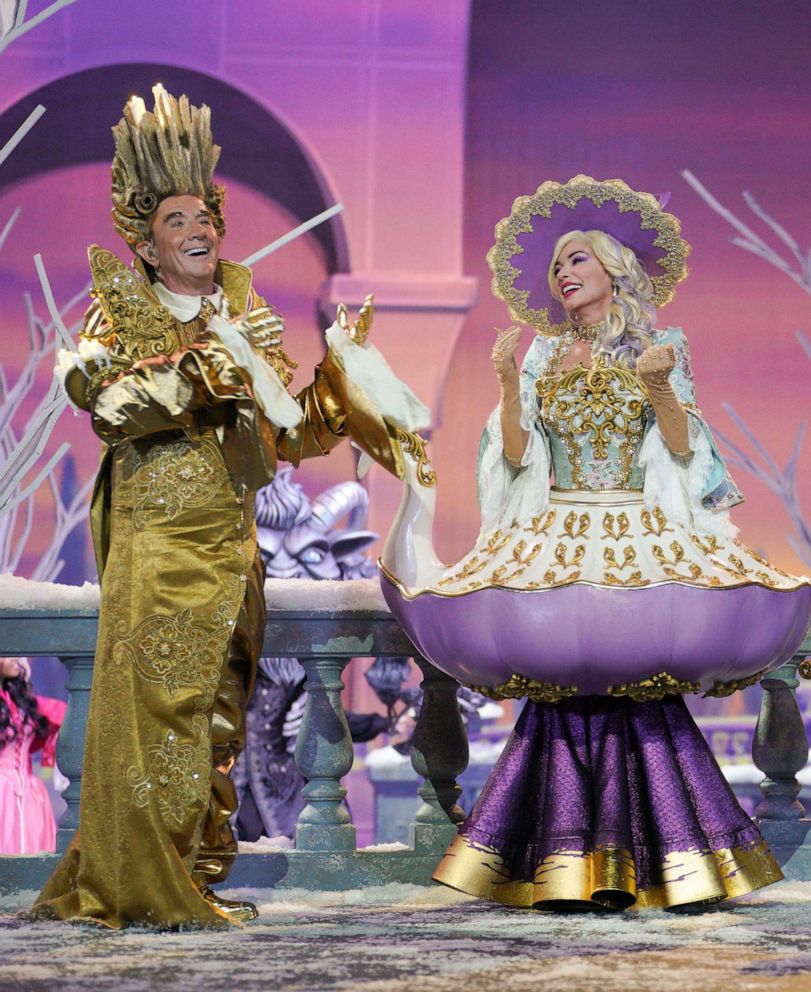The image depicts Martin Short and Ariana Grande on stage, seemingly performing in a production of Beauty and the Beast. Martin Short, portraying the character of Lumière the candlestick, is dressed in an opulent gold suit with golden gloves, a high frilly collar, and his hair styled straight up with curls. He stands with a friendly expression and his hand raised. Beside him, Ariana Grande, embodying Mrs. Potts the teapot, is adorned in an elaborate costume that includes a purple and gold hat, a gold-embroidered purple dress with a flared skirt, and loose white sleeves with frilly cuffs. She smiles brightly towards Martin Short. The vibrant background features hues of purple, pink, blue, and white, creating a fantastical and vividly lit setting perfect for the colorful and clear staging of the scene.